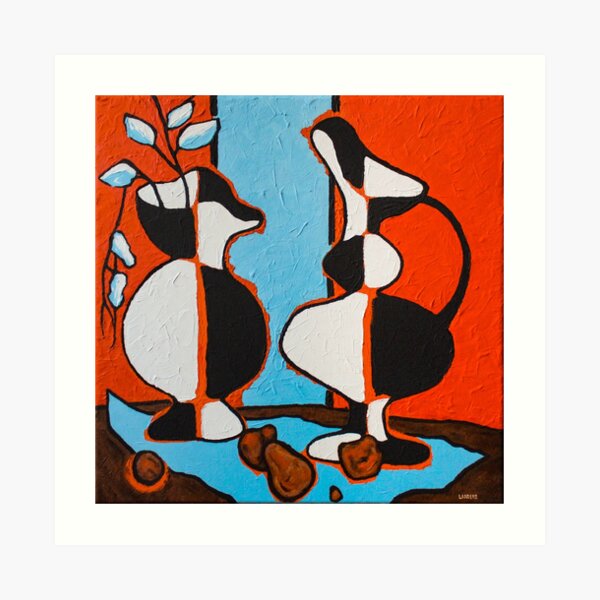The painting is a vibrant and whimsical modern art piece featuring two checkerboard-patterned vases, each with alternating black and white sides. The vase on the left, which has a handle, holds two branches with blue leaves, while the vase on the right, characterized by an hourglass shape with an additional curve on top and an open lip, stands empty. Both vases rest on a brown table covered with a blue square cloth. Scattered between the vases are pear shapes, adding to the eclectic composition. The background features three vertical stripes—red, blue, and red—framing the scene with a bold and graphic presence, enhanced by thick impasto paint and red outlining lines.